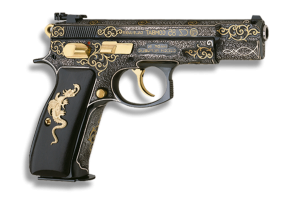This image showcases an exquisite black automatic pistol, accentuated by intricate gold designs. The firearm, likely a nine-millimeter, is adorned with elaborate gold etchings across the barrel and the handle, featuring a detailed image, possibly of a dragon or gecko, with wings atop and a long tail extending downward. The gun's black body is complemented by a gold trigger and a gold-colored screw located behind the handle. There are gold and green patterns intricately woven into the weapon’s surface, emphasizing its ornate craftsmanship. The pistol, oriented to the right with the handle pointing downward, includes black sights on both the front and rear ends of the barrel. A white circle marks the end of the barrel. The firearm is set against a plain white background, casting subtle shadows that highlight its detailed features. This image likely serves to exhibit the firearm's artistic design, potentially for a sales catalog or display purposes.